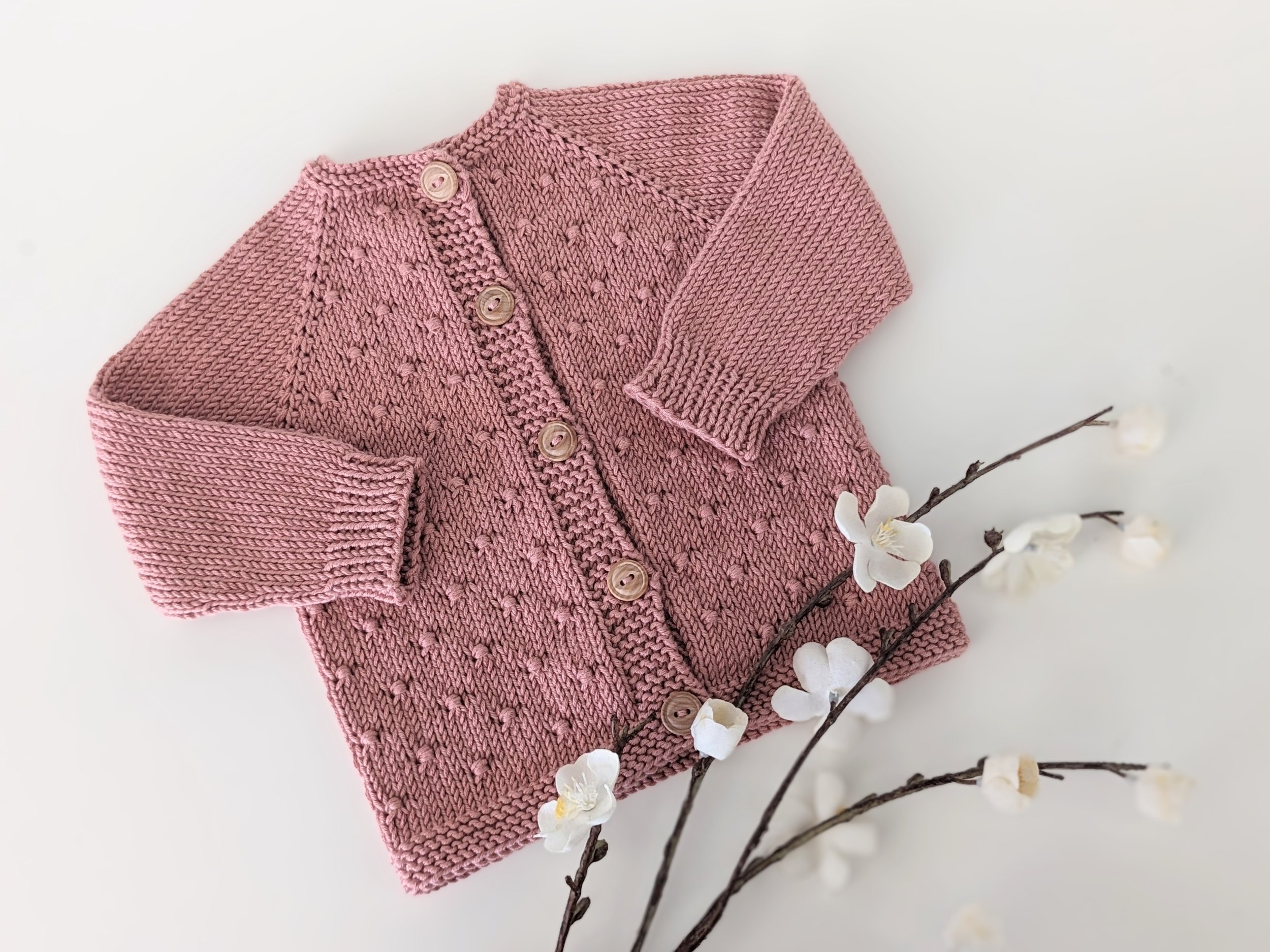The photograph showcases a beautifully knitted, small sweater, likely intended for a child. The sweater is crafted from a muted raspberry yarn and features long, raglan-type sleeves that are thoughtfully folded across its sides. It has a ribbed knit bottom and an edging around the neckline, with five prominent tan buttons that run down the front. The front of the sweater is meticulously detailed, with aligned nubs of yarn enhancing its texture. This charming sweater rests on a backdrop with a grayish-blue, purplish hue, almost violet. Complementing the sweater, at the bottom, are four brown branches adorned with white flowers in various stages of bloom, adding a natural, delicate touch to the scene.